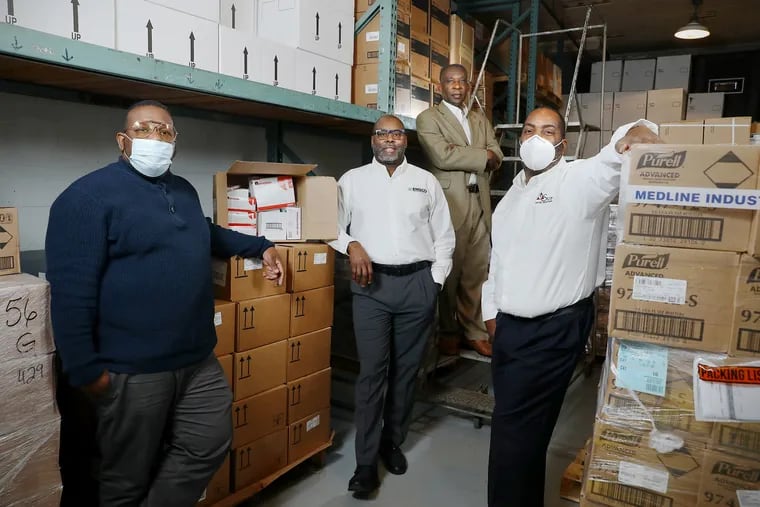The photograph depicts four African American men standing in a well-organized storage warehouse, clearly serving as a distribution center for COVID-19 supplies. The men, all dressed in white dress shirts and dress pants, are positioned around boxes of Purell hand sanitizer and COVID-19 test kits. The detailed scene includes a variety of storage elements such as shelves lined with stacked boxes, a shrink-wrapped pallet on the right, and a rolling ladder in the center background. One man, wearing a dark brown, tan suit, is standing on the ladder, while another, in a blue long-sleeve sweater and gray pants, leans against a stack of boxes that includes an open box revealing its contents. Two of the men are wearing masks: one in a white shirt and black pants with an N95 mask rests his hand on the tall stack of Purell boxes, and another in a blue Henley shirt and gray pants, with glasses, wearing a different style of mask. The man in the center, wearing a white dress shirt and gray pants, leans on one of the boxes on the shelving. They stand proud, seemingly pleased with their contribution, aiding the community's fight against COVID-19 through the distribution of essential supplies.